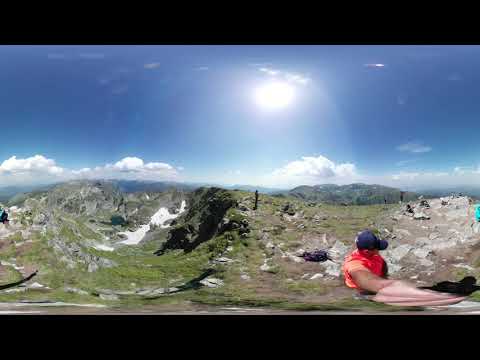The image, bordered by black bands at the top and bottom, captures a panoramic view of a hilly or mountainous terrain during daylight. The upper portion of the photograph showcases a clear blue sky with low-hanging white clouds and the sun shining prominently in the upper middle. The landscape consists of rocky hillsides interspersed with patches of grass. The foreground prominently features a rocky area with grass, transitioning from left to right, with a predominantly rocky section on the far right. 

A person with a blue cap and an orange-red shirt, possibly distorted due to the panoramic effect, stands in the bottom-right corner of the image. They are facing to the right, and their right arm appears stretched out and distorted. The panoramic nature of the photograph stitches multiple views together, creating a curved, almost spherical perspective. This effect results in a second figure in a bright blue shirt, whose image is split and appears both at the very left and very right edges of the picture, suggesting the continuity of the scene if viewed in a spherical format. Overall, the photograph presents a muted yet detailed landscape with scattered human activity, accentuated by the striking natural scenery and clear daylight sky.